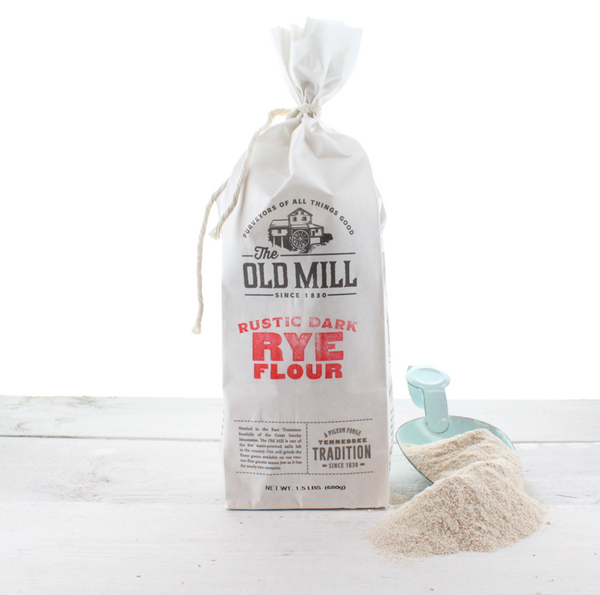The image shows a centered, rustic white (light gray) wooden table with a white sack of The Old Mill Rustic Dark Rye Flour. The sack is tied at the top with a white cord. The packaging features an illustration of a traditional wooden mill and the brand name, "The Old Mill," in black text. Below, in red text, it reads "Rustic Dark Rye Flour." The bottom of the sack mentions "A Pigeon Forge, Tennessee Tradition Since 1830" and notes the net weight of "1.5 pounds." To the right of the sack, a light blue scoop lies on the table with a generous amount of off-white, finely ground rye flour spilling out. The background is a lighter white, highlighting the product and its presentation on the table.